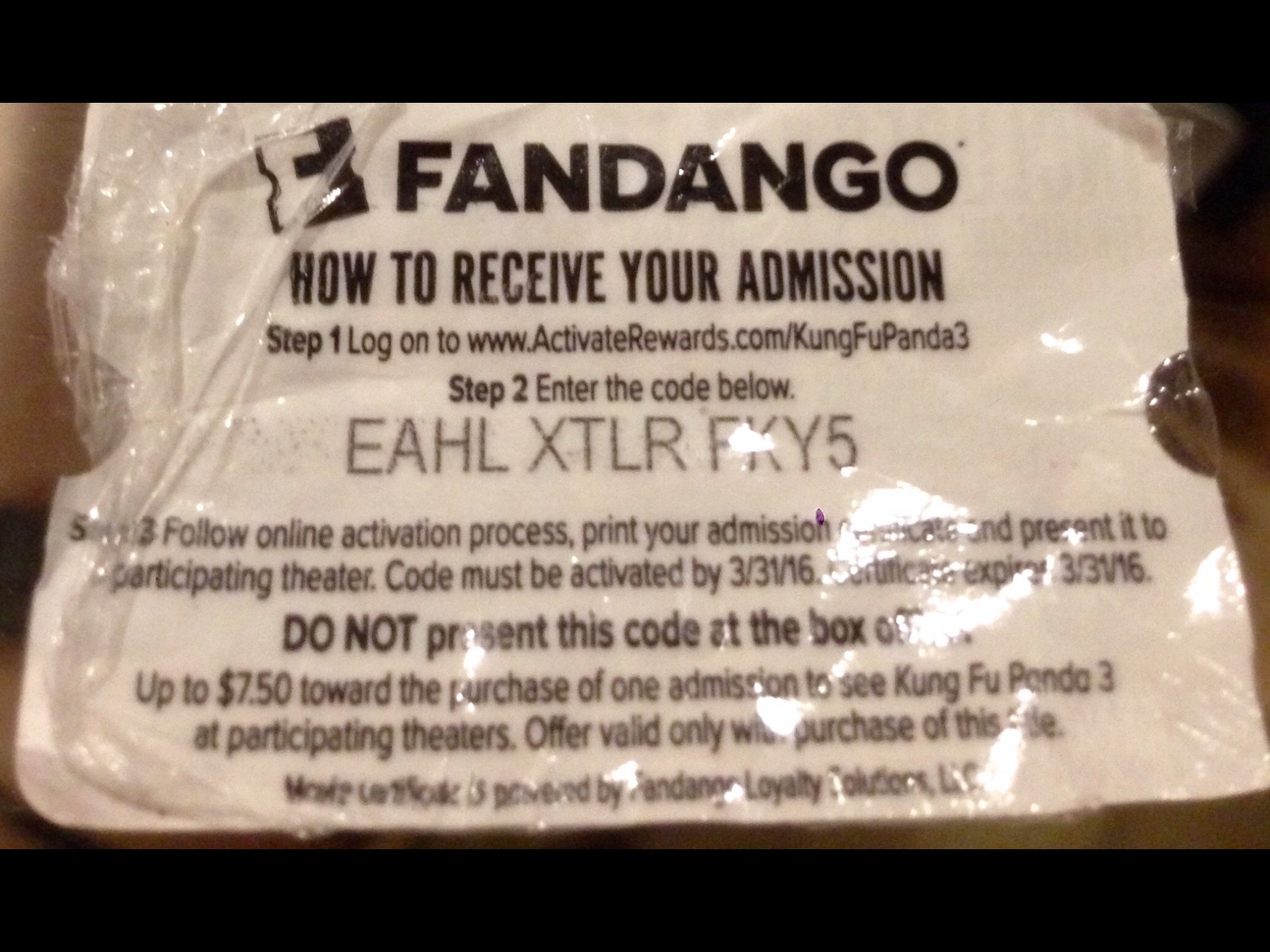In a horizontally oriented rectangular frame, the image displays Fandango instructions for obtaining a code to access an event. The instructions are presented on what appears to be a paper ticket wrapped in plastic or saran wrap, contributing to noticeable light reflections, particularly on the bottom right. The ticket itself is designed to mimic an admission ticket, complete with semi-circular notches on the left and right edges. 

Centered at the top in bold, uppercase letters is the Fandango logo, which includes a white 'F' symbol next to 'Fandango™'. Below this, in all caps, the text reads "How to receive your admission." Following this are three steps:

1. "Step 1: Log on to www.activaterewards.com/KungFuPanda3" (with the first letters of each main word capitalized).
2. "Step 2: Enter the code below – EAHL XTLR FK or XY5."
3. "Step 3: Follow online activation process, print your admission, and present it to the participating theater."

A warning below the steps states, "Do not present this code at the box office."

Additional details explain the offer: "Up to $7.50 toward the purchase of one admission to see Kung Fu Panda 3 at participating theaters. Offer valid only with purchased admission ticket."

The entire instructional label, featuring mixed uppercase and lowercase text, is printed in white on a black background. The package rests on a table, with the image capturing the crinkling of the cellophane in the upper left, adding texture and depth to the scene. The instruction must be activated by March 31, 2016.